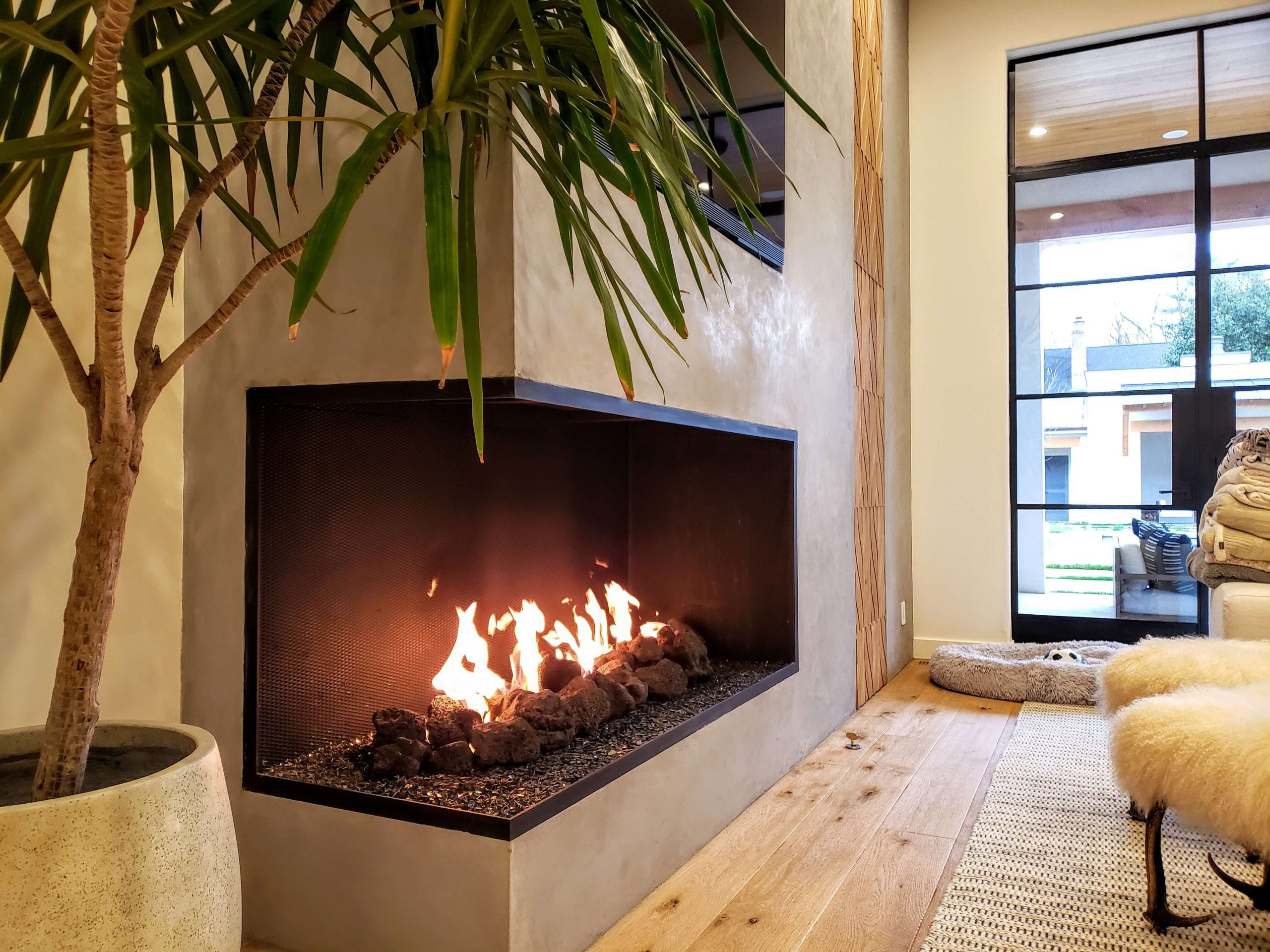This image depicts a serene and stylish living room centered around a rectangular, built-in gas fireplace with medium-height flames, set within a wall of earthy cream and tan shades. The room has a light, modern decor palette dominated by beige tones and earthy creams. On the left side of the fireplace stands a large cream pot with a leafy plant, adding a touch of greenery to the space. A large window with black trim illuminates the room with natural light. The floor is adorned with horizontal wood planks and a wicker-like cream rug, enhancing the room’s cozy ambiance. To the right of the image, partially cut off, is fuzzy white furniture, likely fluffy ottomans, and a gray dog bed with a soccer ball toy. Folded blankets are visible in the background, completing this tranquil and tastefully curated home interior.